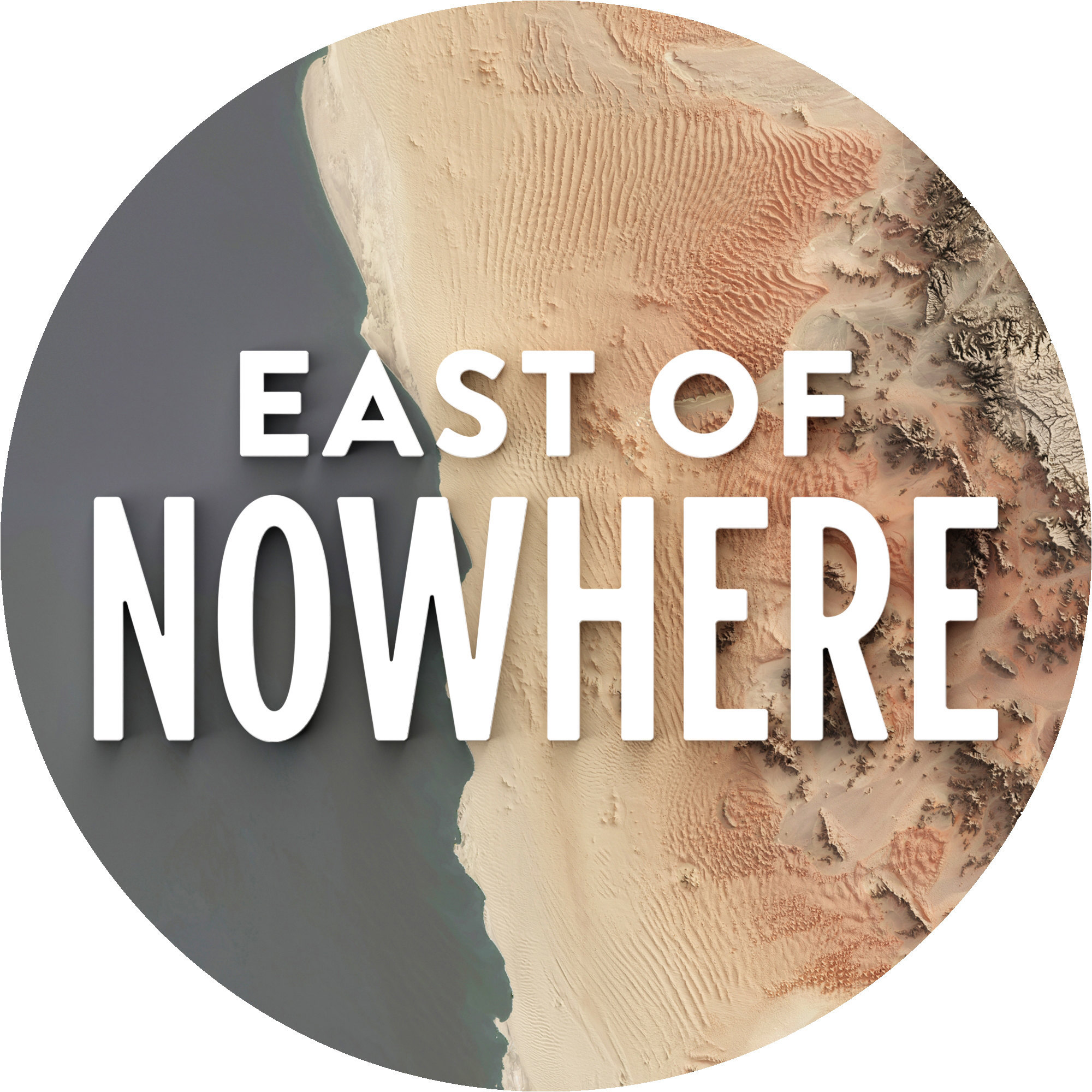The image is a circular aerial view likely taken from a high altitude, perhaps even from space, depicting a coastal desert environment. The left side of the image features what appears to be a vast expanse of grayish-blue water, possibly an ocean. The right side transitions from beige sandy dunes with noticeable ripples and small dunes into areas with darker browns and grays, which seem to represent cliff faces and small mountains, or rocks. There's significant texture differentiation between the water and the varied landforms. The overall coloring is muted, making it difficult to discern finer details, but it could evoke an African coastline or a coral reef.

Prominently displayed across the center of the image is large bold white text that reads "EAST OF NOWHERE" with 'east of' on the first line in smaller text and 'NOWHERE' on the second line in larger text. This bold lettering stretches almost entirely across the circular image, adding a stark contrast to the natural scenery depicted below. The entire image is set against a white background, with no visible people or buildings, emphasizing the desolate and remote feel of the landscape.